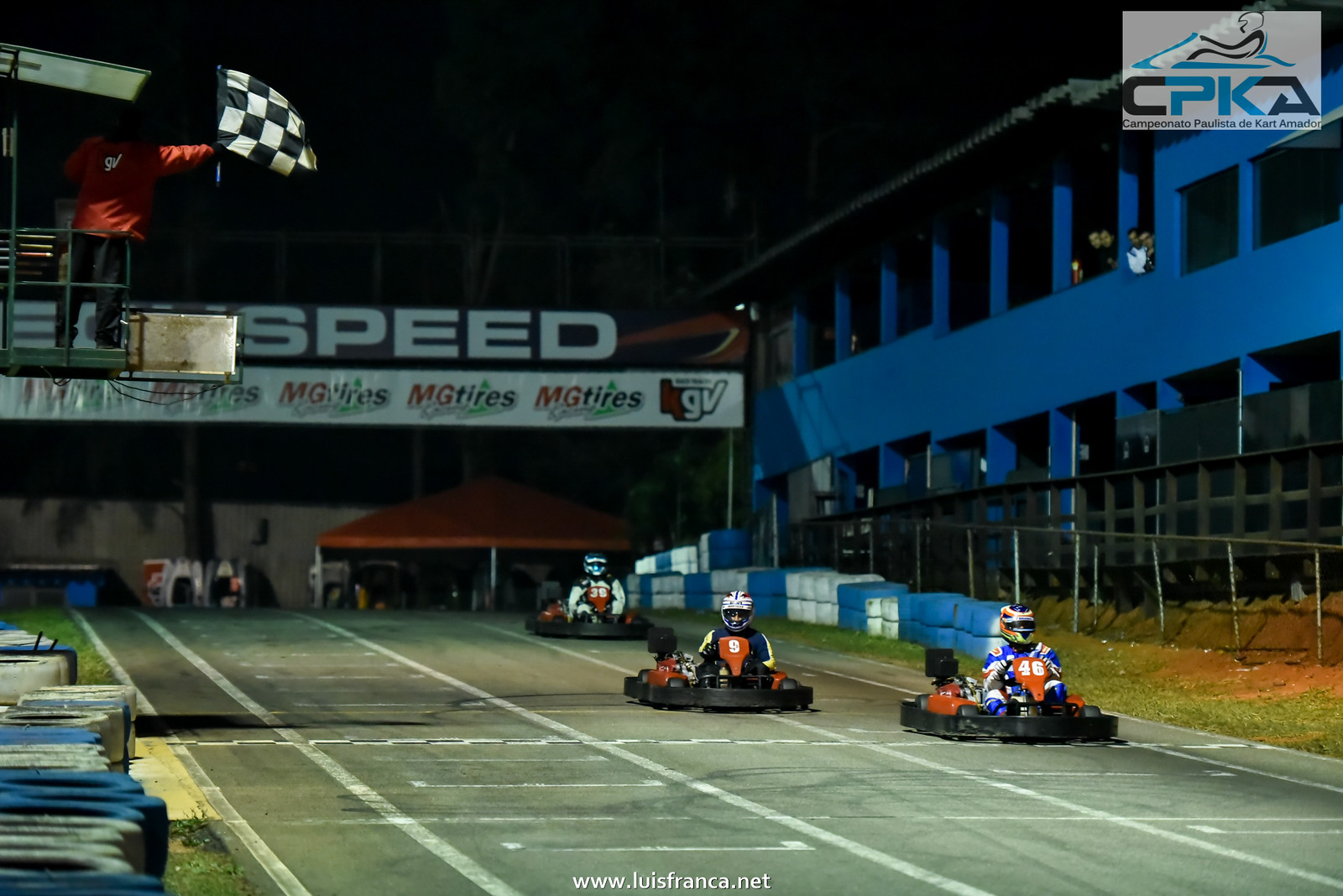The image depicts an exciting night-time go-kart race on a well-lit track with defined white lane separators. The track stretches across six lanes, and the focus is on three go-karts racing towards the finish line. A man in a red jacket and black pants stands on a platform about 20 feet above the ground, poised to wave the black and white checkered flag. The leader, driving an orange go-kart with the number 46, is clad in a blue leather racing outfit and a helmet featuring black, orange, and neon green colors. Trailing him is the number 9 go-kart, also orange, driven by a racer in a dark blue suit with a distinct yellow line running down the sleeves. The third-place racer, numbered 30, maneuvers a black go-kart and dons a blue and white helmet with a white and red racing suit. The background reveals a red canopy area, likely bustling with race officials or spectators, while a blue building with expansive windows stands to the right, allowing a clear view of the intense competition below. Additionally, overhead signage reads parts of "SPEED" and mentions "MG tires," adding to the atmosphere of high-powered racing excitement.